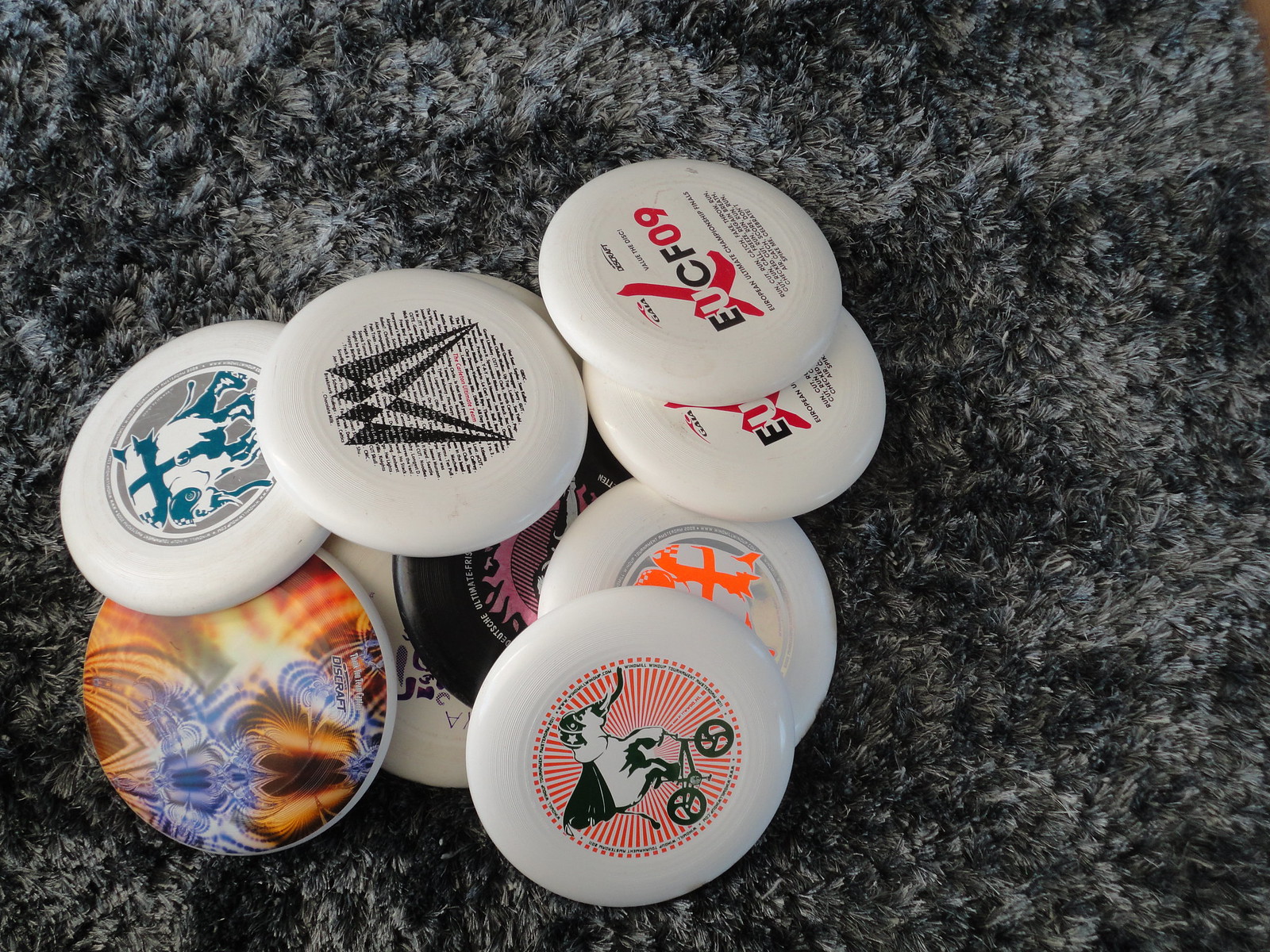In this color photograph, the focus is a slightly off-center pile of frisbees arranged on a plush, multi-toned gray shag carpet with patches of black. The frisbees are stacked, obscuring some designs, but a variety are clearly visible. Predominantly white, they feature circular designs around plain white borders. One frisbee in the forefront showcases a whimsical black and white elephant riding a bicycle. Towards the back, two frisbees have diagonal text reading "EUCF09" in black, white, and red. Another frisbee displays a black triangular (almost W-shaped) design amidst dense text. There are also vibrant designs, such as an abstract pattern in purple, yellow, and red, and another with blue shapes and red and yellow rays. Among these colorful discs, partially hidden, is a black and pink frisbee, and another with a blue and white elephant with a tusk and an object strapped to its back.